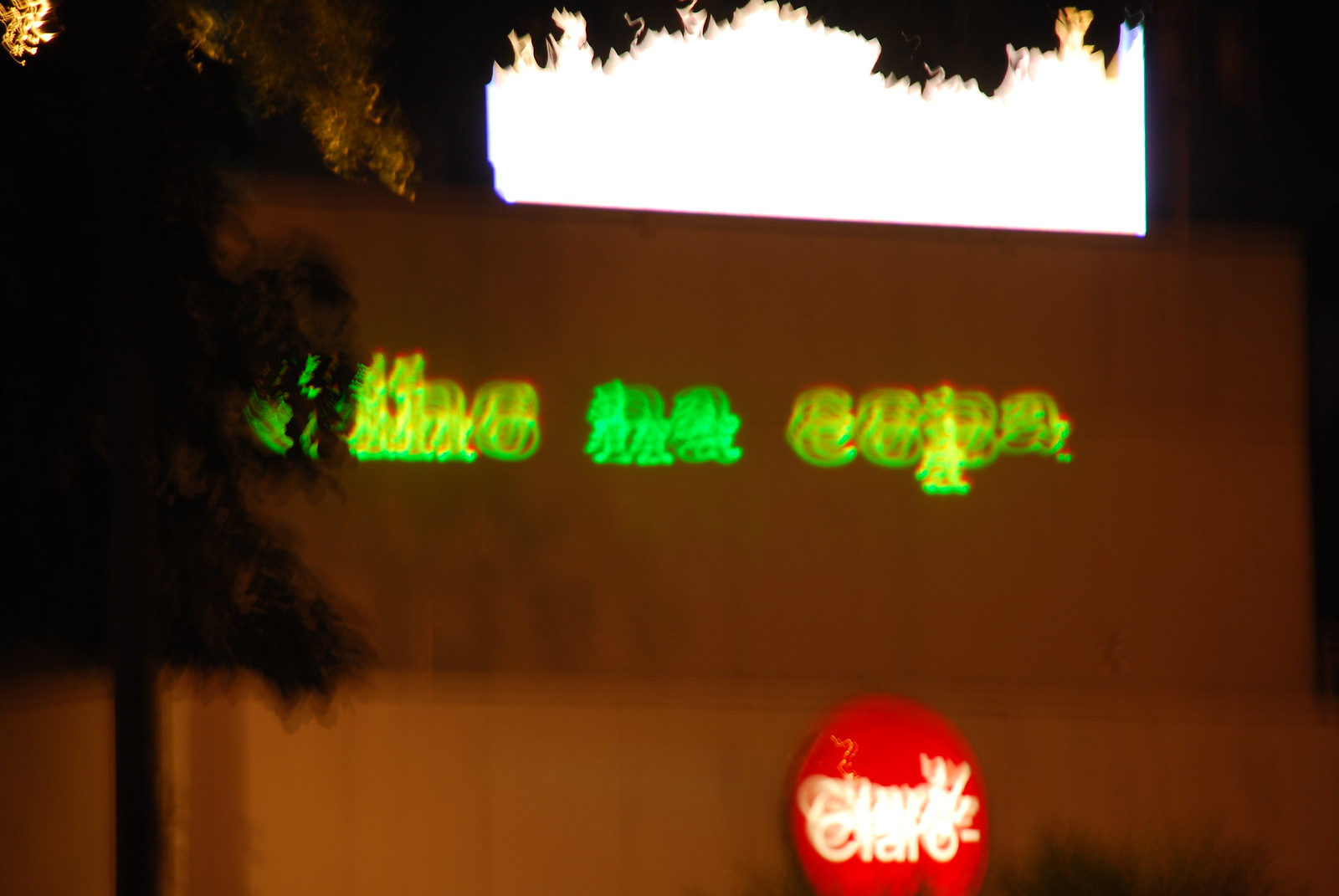The image captures a nighttime scene with a very blurry, out-of-focus snapshot of the front of a restaurant-like building. The building appears square and low, possibly made of yellow or tan bricks. Dominating the top portion of the scene is a large, illuminated, bright white rectangular sign, possibly mounted on the roof, which is empty or too bright to display any visible text. 

In the center of the building façade, three neon illuminated words in a greenish-yellow hue stretch across. Due to the blurry double-image effect, the exact wording is indecipherable, although there is speculation that one word may be "Copa" and another might contain the letters "NA." 

Near the bottom right of the photo is a red circular sign with white lettering, also affected by the blurriness, making the text appear as though it is repeated several times, and possibly spells out "CIARO" or something similar.

The left side of the image features the silhouette of a tree with branches hanging down and partially obscuring the sign. The upper middle of the image includes either a white light or an empty patch of sky, contributing to the overall indistinctness of the scene.